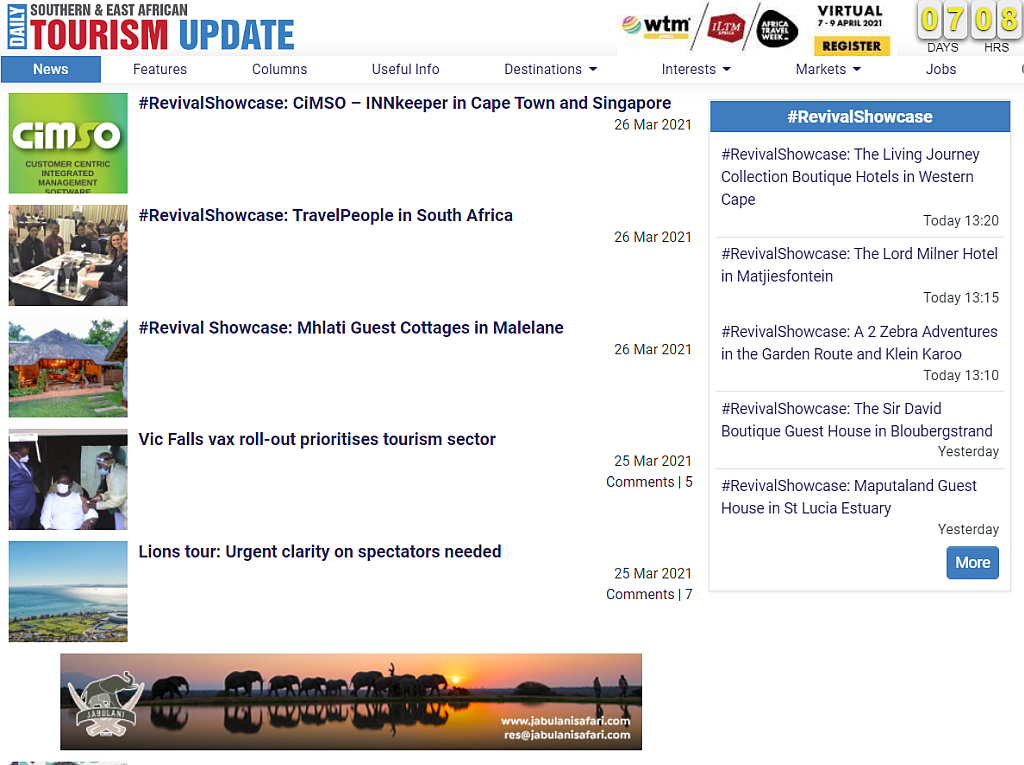The image showcases a webpage from the Daily Southern and East African Tourism Update. In the upper left corner, the website's name is prominently displayed in bold font, with "Tourism in Bold" written underneath, accompanied by readable update information highlighted in blue. On the upper right side, there is a timestamp indicating "7 days, 8 hours."

To the left, there is a virtual event mentioned, scheduled for 7-9 April 2021, with a yellow action button labeled "Register."

The navigation bar, from left to right, lists the following sections: "News" (highlighted in blue), "Features," "Columns," "Useful Info," "Destinations" (with a pull-down menu), "Interests" (with a pull-down menu), "Markets" (with a pull-down menu), and "Jobs."

Beneath the "Jobs" section, under the hashtag "Revival Showcase," there are three highlighted events:
1. "The Living Journey Collection Boutique Hotels in Western Cape, today 13:20."
2. "The Lord Milner Hotel and Match v. Spontine, today 13:15."
3. "A Two Zebra Adventures in the Garden Route and Klein Karoo, today 13:10."

Each event appears to be listed with the hashtag #RevivalShowcase, providing specific details and times for today's schedule.